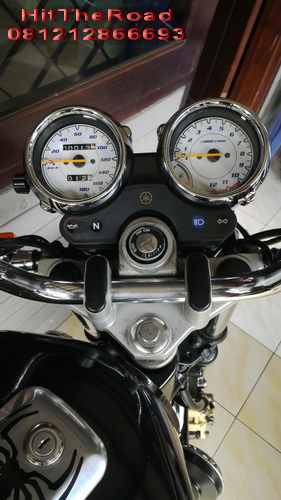This detailed caption provides a vivid description of the scene:

"Close-up view of the handlebars and instrument cluster on a motorcycle, possibly a moped or a motorized two-wheel vehicle. The handlebars are turned approximately 45 to 60 degrees to the left, showcasing the silver crosspiece and the connecting bolt that secures the front end of the bike to the frame. The ignition key is visible above the silver bolt, encased in a small black console with illuminated indicators for high beams, neutral gear, and other functions.

In the center, two chrome-encased gauges with white faces stand out. The left gauge is a speedometer with blue markings and an orange needle, while the right gauge appears to be a tachometer, marked from 1 to 12 in increments of 1,000 RPM, also featuring an orange needle. 

In the upper left corner of the image, the text 'hit the road 08-121-2866693' is displayed, suggesting a possible phone number, potentially from a foreign country. The detailed arrangement and clear view of the components highlight the sophisticated design and functionality of the vehicle's dashboard."